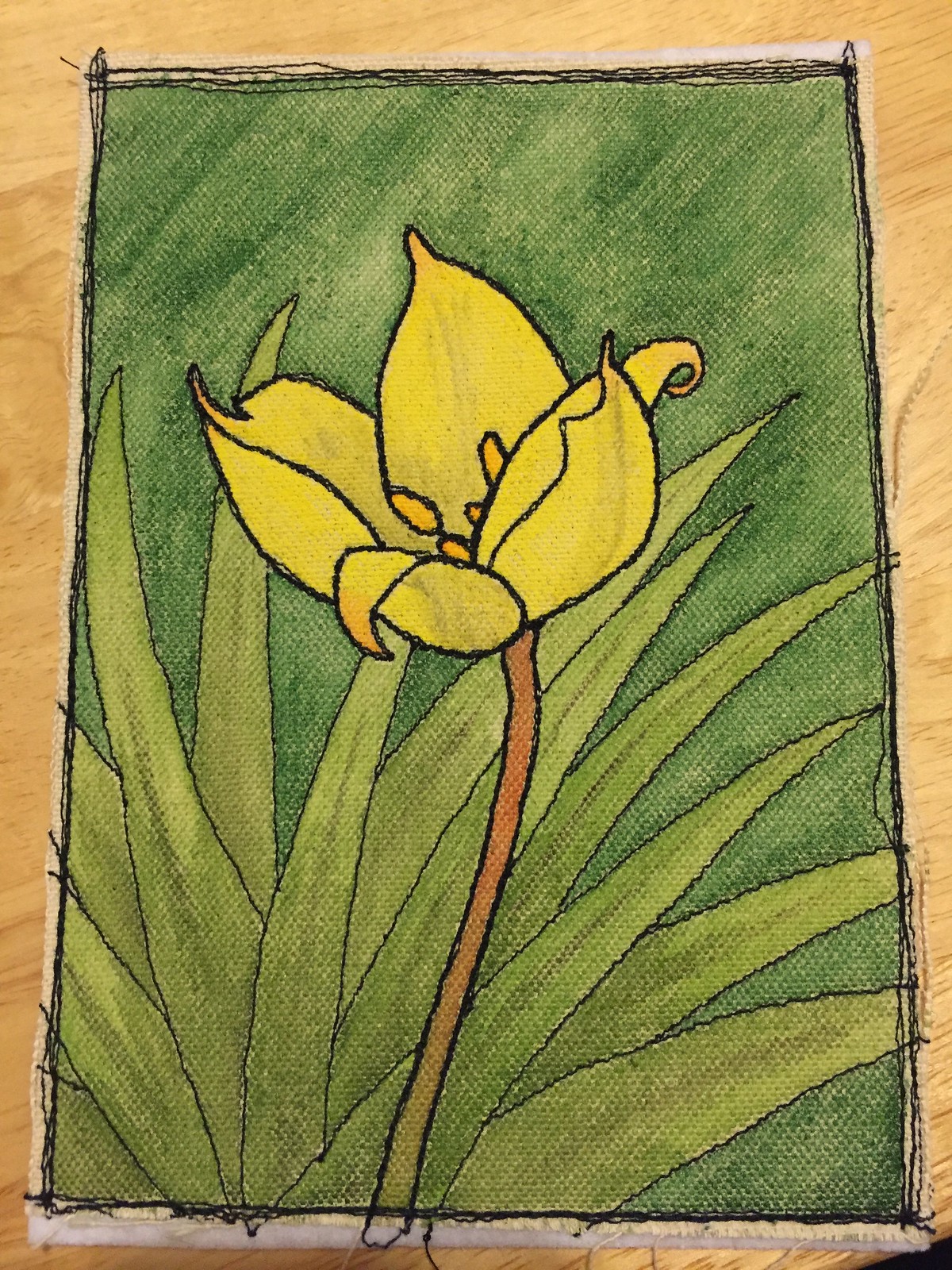This image is a detailed photograph of a fiber art piece depicting a tall yellow flower, which appears to be a tulip, with intricate design elements. The flower is distinguished by its four yellow petals, accented with orange flower pieces inside, mounted on a brownish stem. This art piece is on canvas, fastened to a wooden frame, and set upon a light brown wooden surface. The background of the artwork features various shades of green, possibly representing a green fern or aloe leaves, adding depth and texture to the composition. The entire art piece, including each element of the flower, is meticulously traced with black thread embroidery, giving it a defined and handcrafted appearance. The canvas is bordered by a dark green or black painted edge, further emphasizing the central floral subject. The image exudes a natural and artistic aesthetic with no textual elements, the focus solely on the handcrafted and painted flower set against its rich, green background.